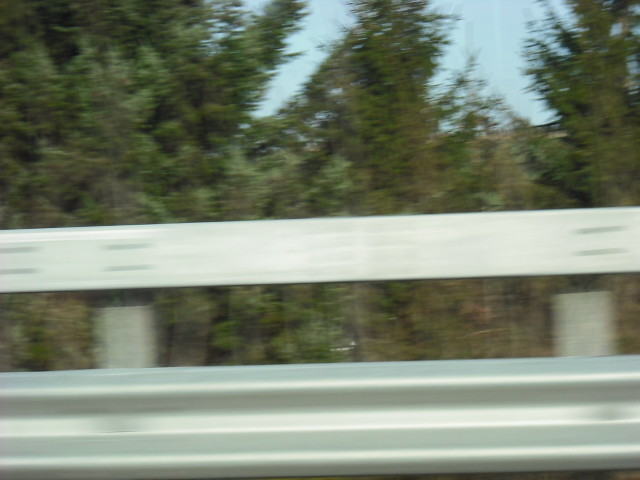This is a blurry photograph captured from a moving car. Dominating the bottom of the image, a silver guardrail stretches across the width, consisting of two beams - one at the base and another in the middle. The middle beam is aligned along the center of the photograph. Behind the guardrail, numerous trees stand tall, their green leaves indicating a summertime scene, with some leaves showing a hint of brown. At the top, clusters of leaves partially obscure the view of the bright blue, slightly overcast sky, which peeks through gaps between the foliage.